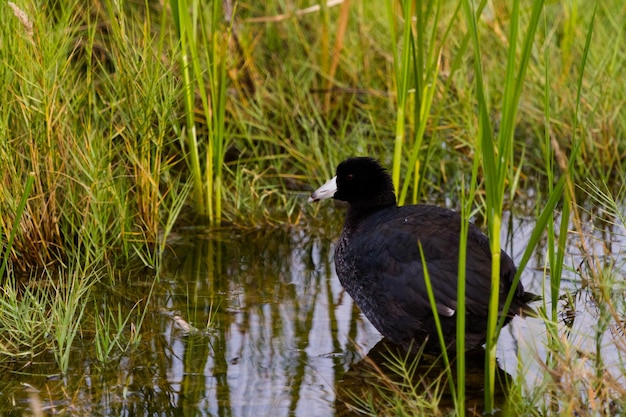The photograph features a large black waterfowl with a white beak and beady black eyes, likely a duck or similar species, positioned slightly right of center towards the bottom of the image. The bird, with dark gray and mottled feathers, is standing on a rock surrounded by patches of green grass and various weeds. The foreground and background are dominated by abundant water, possibly a small pond with reflections of the sky, while the left side showcases additional vegetation, including grass and weeds both in and around the water. Tall green grasses, reeds, and brush fill the upper portion of this horizontal, rectangular image, enhancing the natural and serene setting of what appears to be a swampy area.